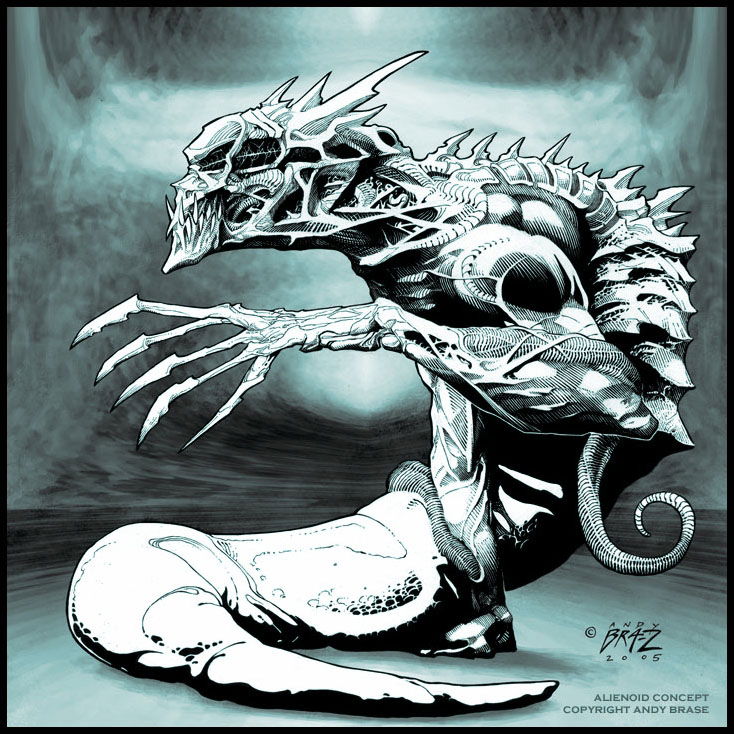This intricately detailed computer-generated cartoon image, copyrighted by Andy Braz in 2005, depicts a fearsome alienoid creature. The alien, drawn in shades of black, white, and greenish-gray, faces to the left in a crouched, pouncing position. It features a long, snake-like tail that twists from the left around to the bottom right, where the copyright text reads "Andy Braz, 2005. Alienoid Concept." The armor plating on its breast and back adds to its menacing appearance. The alien's upper body, resembling a human, contrasts sharply with its lower body, which mimics a large tail. Its head is adorned with horn-like protrusions, including one notably longer horn in the third position from the front. The face, reminiscent of a skull, houses sharp teeth and is intricately detailed with fine lines. The creature's left arm is raised and pointed to the left with razor-sharp claws extended, while its right hand supports its twisted body on the ground, adding to the overall menacing and predatory stance.